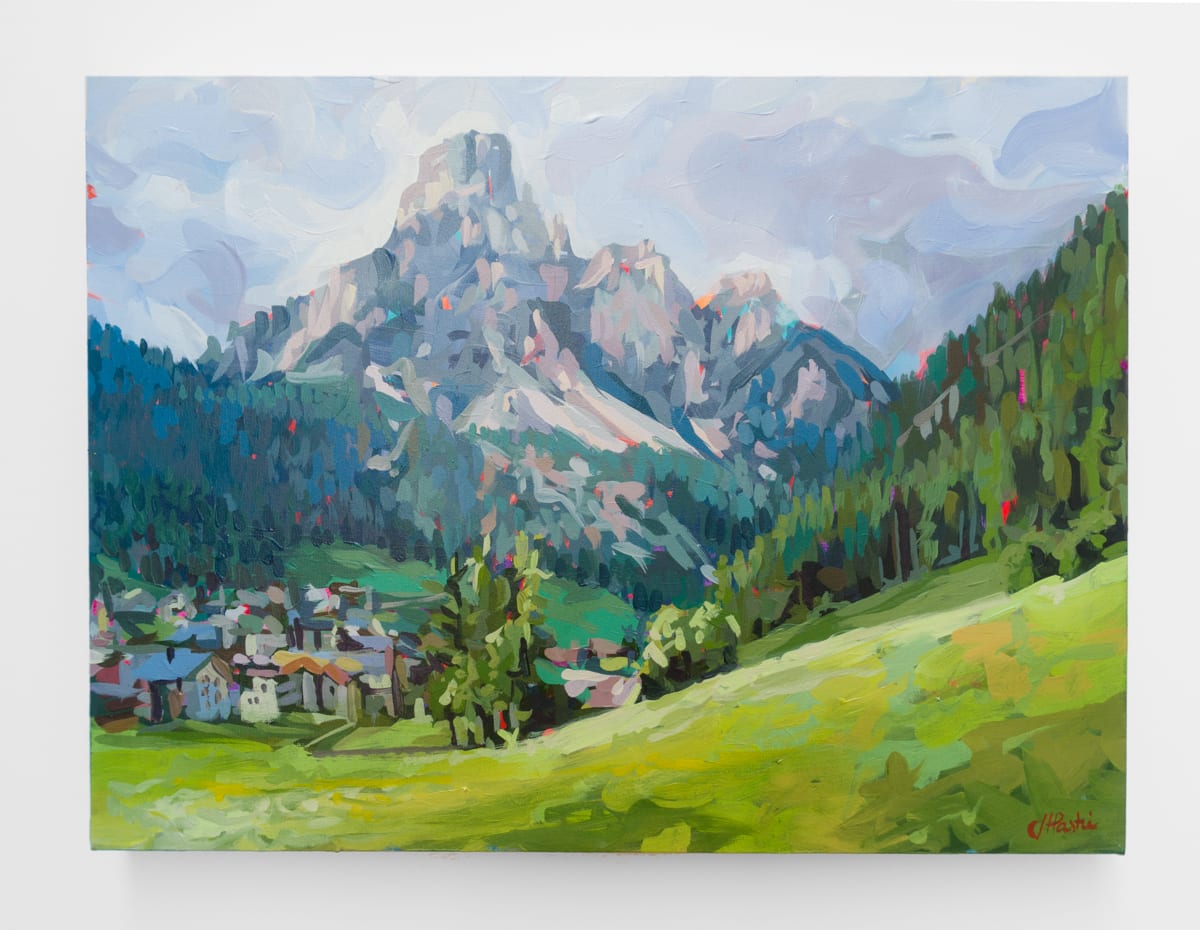The artwork is a detailed painting depicting a picturesque mountainside scene. At the top of the image is a towering, hilly mountain painted in shades of white, blue, and green, with hints of snow on its peaks. The sky above is textured with blue hues and scattered clouds, becoming darker around the edges. In the foreground, the hillside is lush with various shades of green and textures, giving life to trees that have blue and green tones, with some red textures interspersed, particularly on the right side.

Nestled below the mountain is a vibrant village with houses of many colors, including orange, blue, purple, pink, green, and gray. The roofs are colorful and varied, and the houses themselves are less detailed, giving an abstract feel to the village. On the left side of the village, the slope is covered in green grass mixed with touches of yellow. 

On the bottom right corner, there is a signature of the artist, though it's not clearly legible. The whole piece is framed in white, enhancing its presentation. The scene evokes the charm of a European hillside village, reminiscent of settings in places like Switzerland, making it an impressive and captivating piece of art.